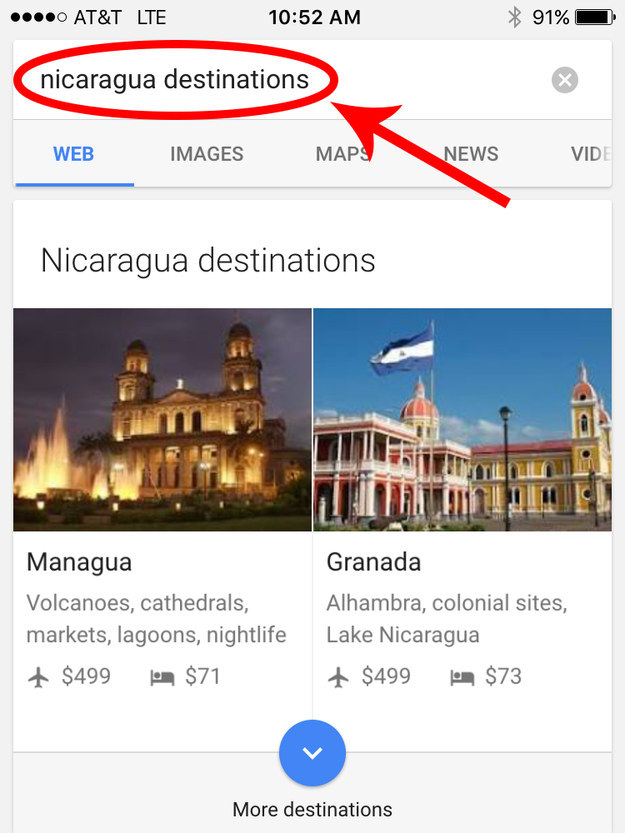This mobile screenshot, captured at 10:52 a.m., displays a search query for "Nicaragua destinations" on the AT&T LTE network with a signal strength of four out of five bars. The battery is at 91% and Bluetooth is enabled, as indicated by the icons on the top right corner. A search bar is visible below the status icons, featuring the text "Nicaragua destinations" circled in red, with a red arrow pointing to it. 

Currently, the search is set to the "web" category, which is highlighted in blue and underlined. 

Following the search options, a white box appears showing detailed information. On the left side of this box, there's an image of a grand palace taken at night, featuring two blue domed columns and an ornate design that suggests a presidential building. The surroundings include a large fountain and illuminated lights. This section provides details about Managua, highlighting volcanoes, cathedrals, markets, lagoons, and nightlife, with airfare listed at $499 and lodging at $71.

On the right side of the box is an image of two colorful buildings. The left one is pink and white with a large pink dome, and the right one is yellow and white with a pink roof. A Nicaragua flag waves against the blue sky in the background. This part describes Granada, noting attractions such as Alhambra, colonial sites, and Lake Nicaragua, with airfare at $499 and lodging at $73.